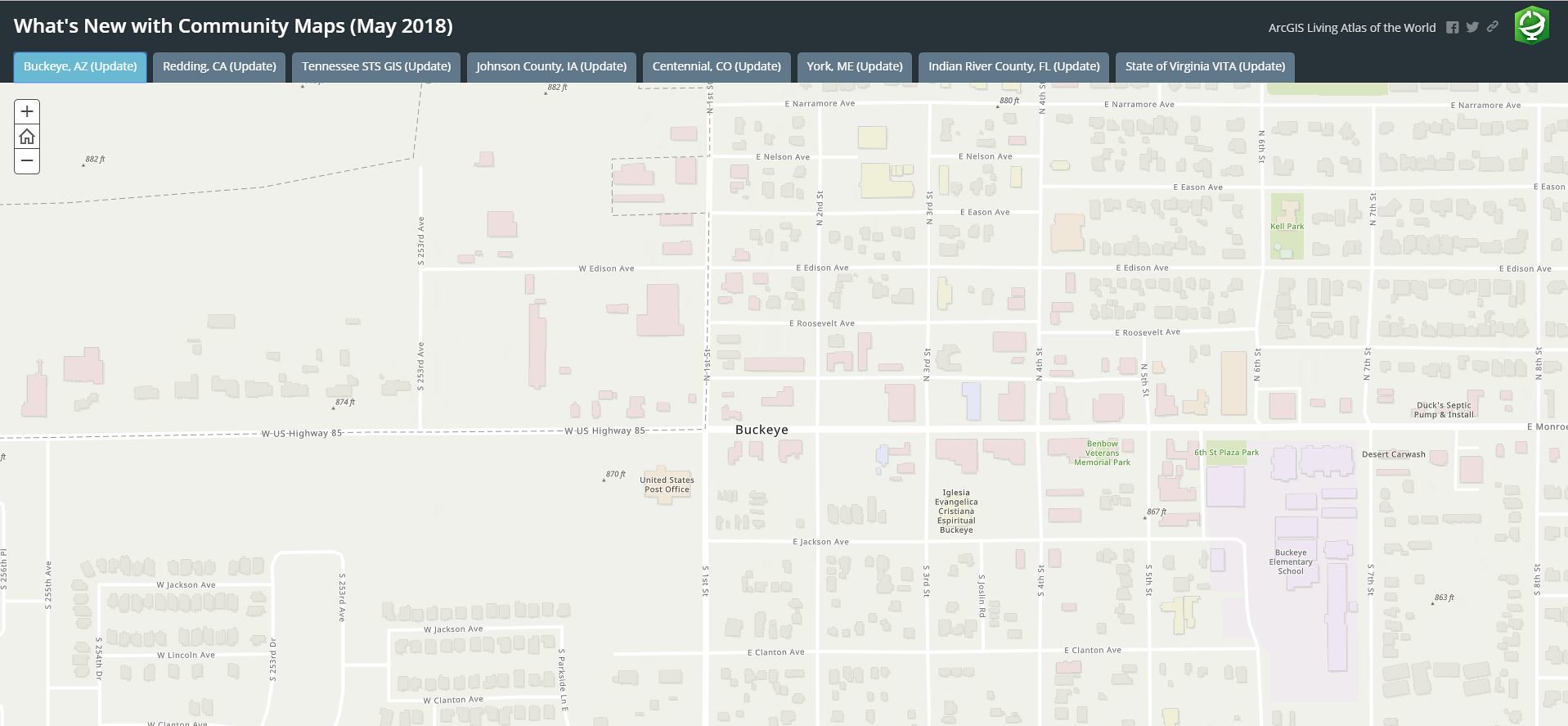This image is a detailed screenshot of a community map showcasing the area of Buckeye, Arizona, as evident from the selected tab. In the upper-left corner, a text box titled "What's New with Community Maps (May 2018)" informs users about the latest updates. Several other locations can be accessed via tabs, including Reading, California; Tennessee STSGIS; Johnson County, Iowa; Sentinel, Colorado; York, Maine; Indian River County, Florida; and the State of Virginia VITA (update).

Central to the map is the town of Buckeye, clearly marked and surrounded by notable landmarks and infrastructure. Prominent highways such as West US Highway 85 are displayed, providing clear routes through the area. To the right side of the image, several key locations are highlighted, including Buckeye Elementary School, Bembry Veterans Memorial Park, and 6th Street Plaza Park. The map meticulously labels every street in the vicinity, adding to the comprehensive layout of this community-focused navigation tool.